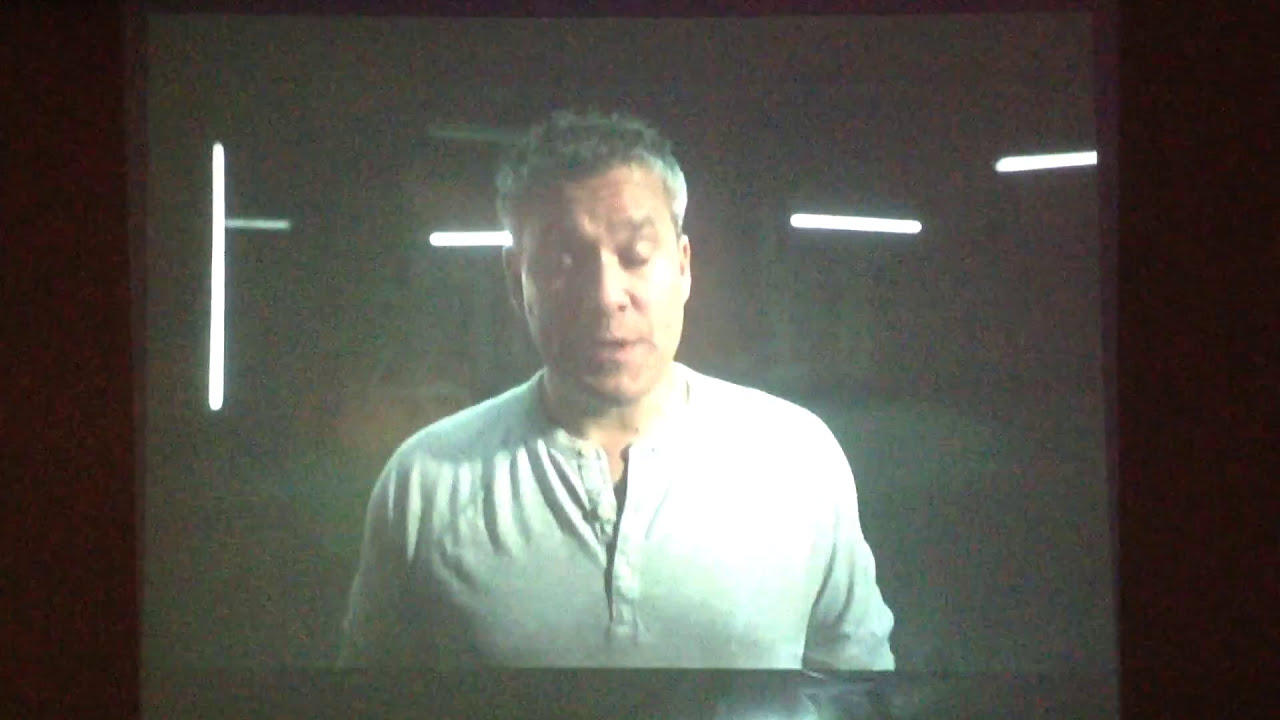The image depicts a middle-aged man, likely in his late 40s to early 50s, captured from the chest up in a somewhat dimly lit setting. He has peach-colored skin and salt-and-pepper hair, spiky and darker on top, graying on the sides. The man is wearing a white long-sleeve shirt that resembles a baseball style with several buttons down to the mid-chest. His gaze is directed downward, and his mouth appears to be mid-speech, suggesting he might be answering a question or giving a speech. The background is predominantly dark, possibly resembling an underground garage or concrete room, with just enough light to distinguish four light bars. Three of these bars are horizontal and positioned behind him, while one vertical bar is over his right shoulder. The overall quality of the image seems low, adding to the ambiguity of the scene's setting.